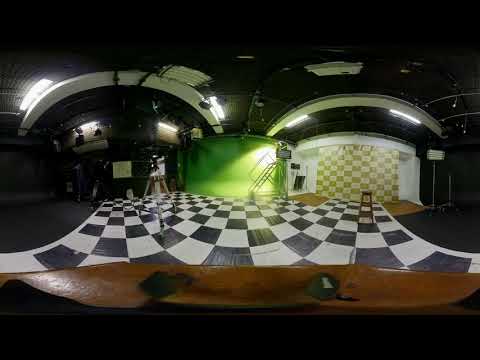The photo depicts a film studio set inside a large warehouse, featuring a black and white checkered floor at the center. Surrounding this central flooring is an area of black flooring. A prominent lime green wall is situated in the background, with a beige and gold checkered wall to its right. On the right side of the image, a stool rests on the checkered floor. Towards the left, a camera tripod is positioned. The ceiling is dark and equipped with hanging lights and an air conditioner, creating a moderately lit environment. The lighting setup above illuminates the set, while additional screens hang around the area. The room is not completely dark, nor is it overly bright. The overall scene is intricately detailed with elements like a domed area and varied wall designs, contributing to the studio's ambiance.